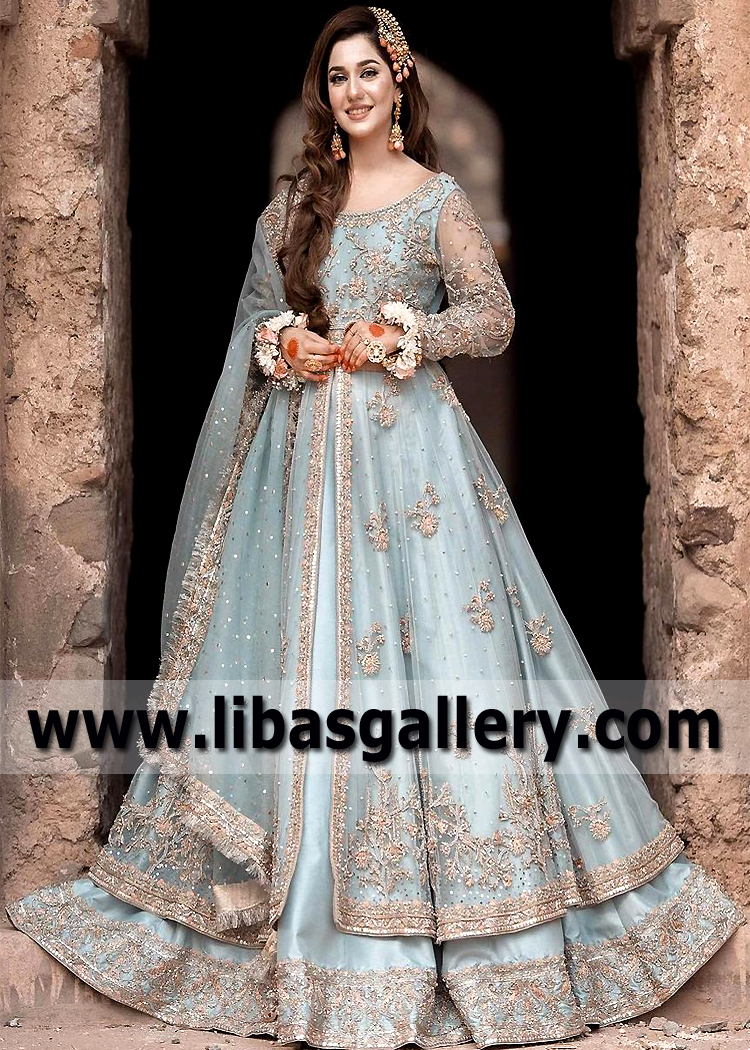A striking photograph captures a woman with long, wavy, dark brown hair, standing gracefully in a doorway made of beige rock, likely part of an old ruin or ancient structure. Her dress, a long, elegant gown in light blue with hints of grey, features intricate gold embroidery and beadwork, enhancing its classy and sophisticated appearance. The gown's sleeves are crafted from a delicate net material, adding to the dress's intricate detail. She accessorizes with a headpiece and large earrings, and her hands are adorned with orange paint. The background has a dark hue, possibly an alleyway or the interior of the ruin, creating a dramatic contrast with her attire. At the bottom, the URL www.libusgallery.com is prominently displayed in black, suggesting where more of this photographer's work can be viewed.